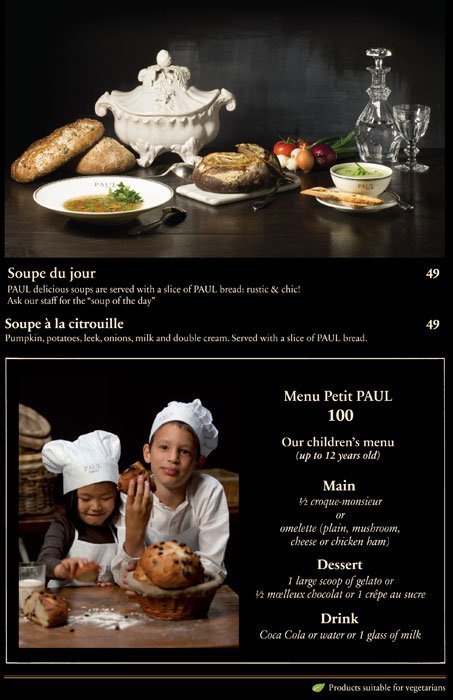This image displays a sophisticated, high-end restaurant menu set against a black background with two main sections, both highlighted by photographs. The top third features a still life fine art image depicting a terrine, a glass of soup, some bread, a crystalline decanter, and a glass, evoking an elegant dining experience. Below the photograph, two menu items are listed: "Soup du Jour" and "Soup a la Citrouille," each priced at $49. 

The bottom section captures a charming photograph of two children in baker outfits—a girl on the left and a boy on the right—standing in front of an array of baked goods; the boy is holding a pastry with chocolate chips. Beside this image, the "Menu Petit Paul 100" or children's menu is detailed in a vertical layout, listing a main course, dessert, and drink in white text. This contrast between the adult and children's offerings underscores the menu's diverse appeal, catering to both sophisticated tastes and family-friendly options.